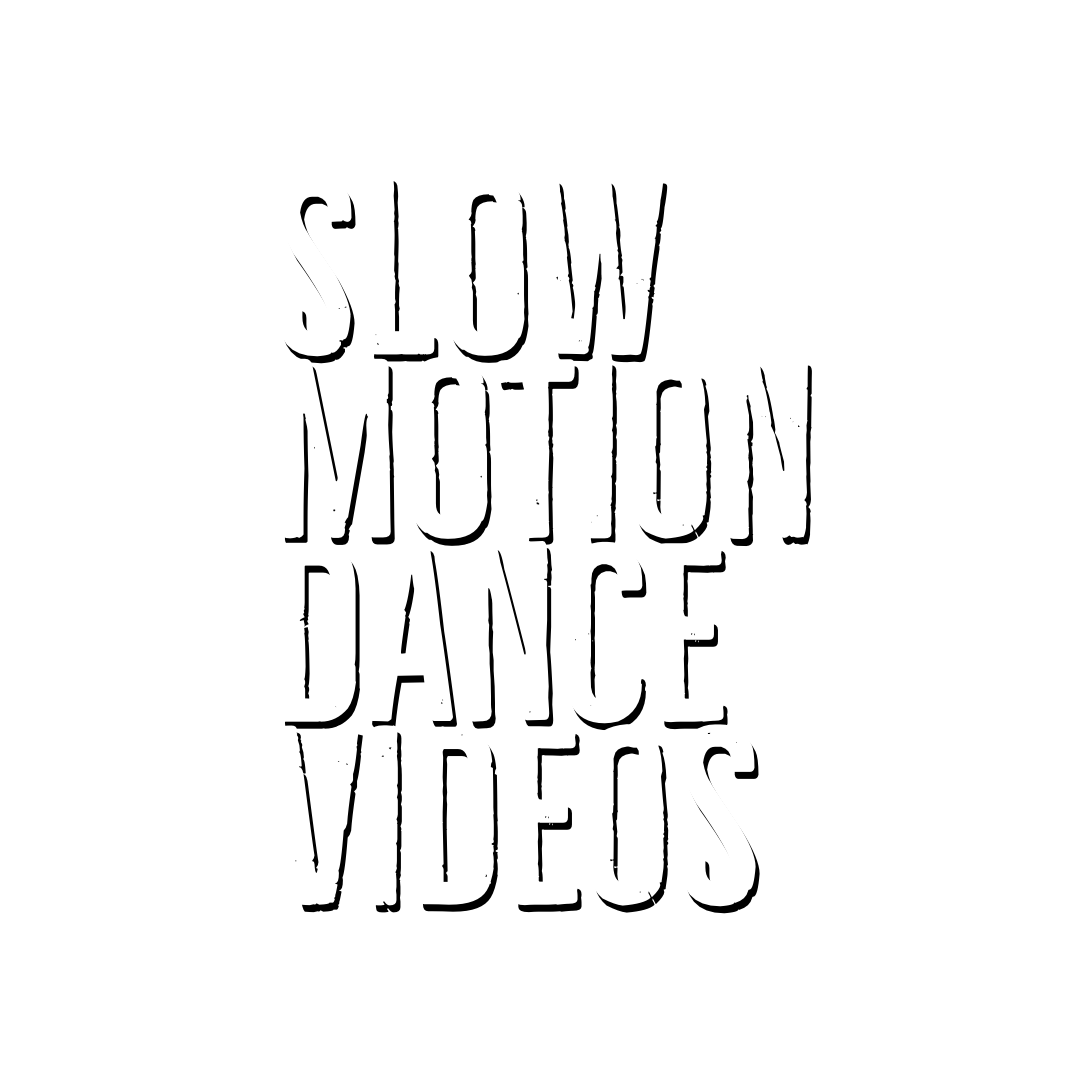The image depicts a close-up of a white poster against a white background, featuring blocky, capitalized text arranged in four lines. The text reads "SLOW" on the first line, "MOTION" on the second, "DANCE" on the third, and "VIDEOS" on the fourth, all aligned to the left edge while the right edge appears irregular and not neatly aligned. The white letters are shadowed in black, creating a 3D effect that makes them appear raised and somewhat indented, giving a worn, slightly beat-up look. The shadows on the right side of each letter enhance this effect, making the text stand out prominently from the background. The poster's minimalist design and stark contrast suggest it is promoting slow-motion dance videos.